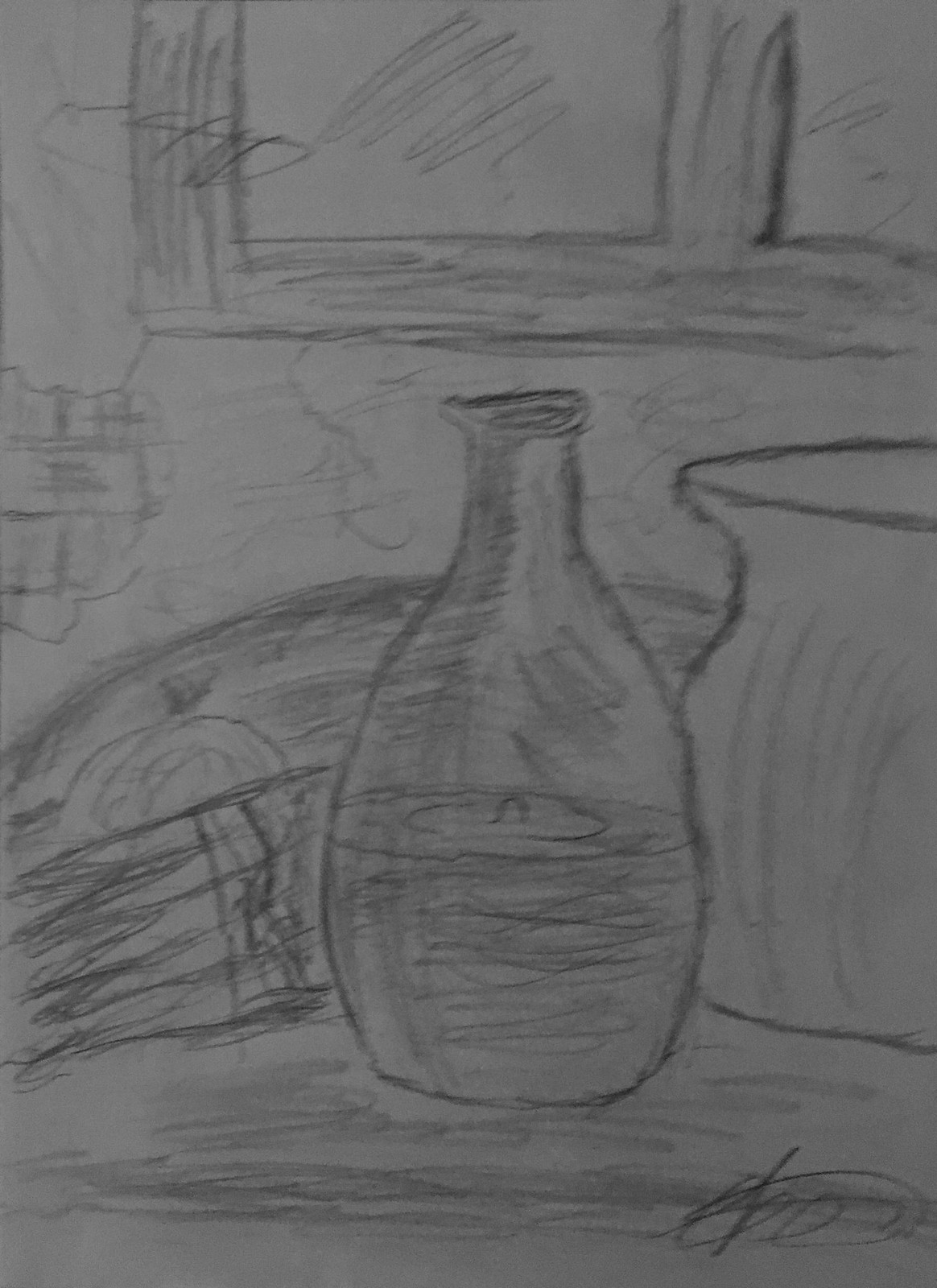This is a detailed pencil sketch, potentially featuring areas of charcoal, depicting a still life of a kitchen worktop scene. Dominating the upper background, there's an old-style wooden window with four panes, adorned with squiggly lines to denote glass and light reflections. Surrounding the window is a wall showcasing uneven textures, some parts appearing as plaster with exposed brickwork where the wall has crumbled away. 

The focal point of the foreground is an oval-shaped bottle or carafe, half-filled with liquid, its narrow neck adding definition. Slightly to its right rests a white pitcher, seemingly empty and finely shaded to show depth. Adjacent to the bottle, on the left, sits a basket of fruits, including a notably round fruit with a tuft of leaves. Further towards the left, a drying rack is noticeable, suggesting kitchen utility. 

All elements of the drawing are rendered in black and white, contributing to a cohesive monochrome aesthetic. The sketch is signed by the artist in the bottom right corner, although the signature remains indistinguishable. The overall composition and use of shading create a vivid, textured scene filled with both practicality and charm.